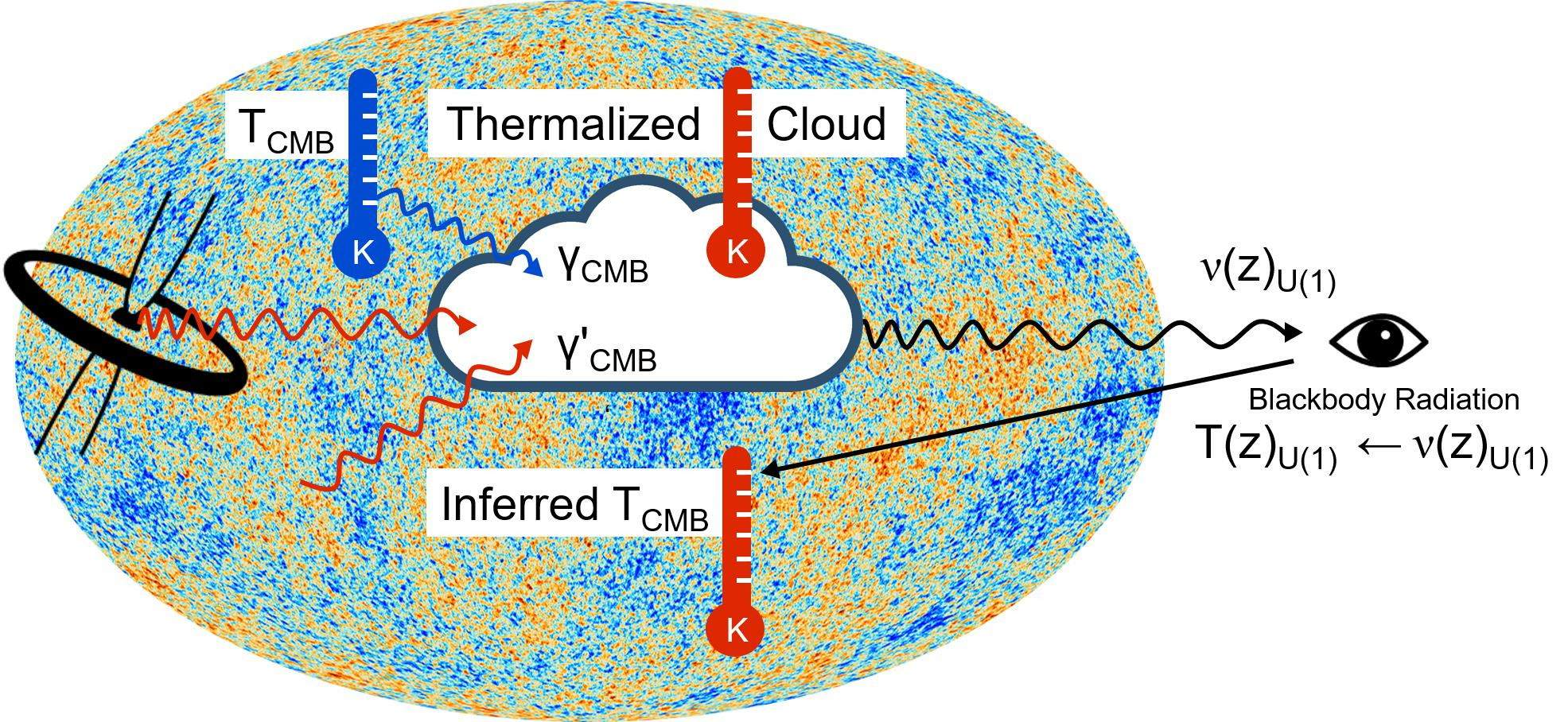The image is a detailed diagram featuring an elongated, egg-like globe depicted in shades of red, blue, and white dots. Central to the image is a "Thermalized Cloud" with a red thermometer marked with "K" indicating Kelvin, and the label "YCMB" and "Y'CMB" on a cloud shape nearby. On the left, a satellite characterized by red squiggly lines connects to this cloud, displaying the interactions of radiations. Above the satellite, a blue thermometer labeled "TCMB" with a K at the base and a blue line connecting back to the cloud is shown. To the right of the globe, an eye symbol labeled "Blackbody Radiation" is connected to the globe with a black squiggly line, near which is the formula V(Z)U(1) and TZ(U)1, V(Z)U(1). Below, another red thermometer is labeled "Infrared TCMB." The diagram intricately illustrates various temperatures and radiations, reflecting on their interactions and the concept of thermal radiation.